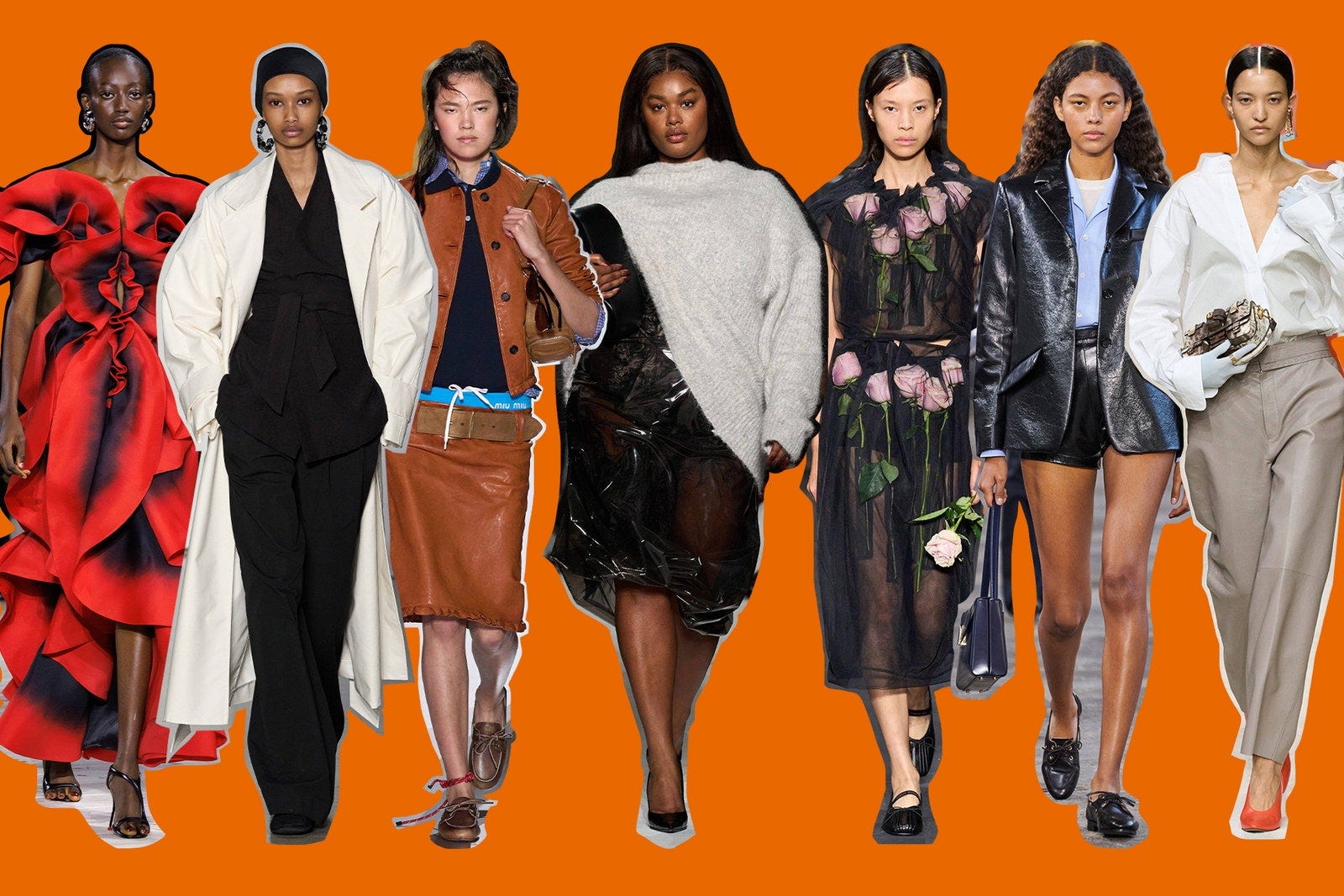The image features seven diverse female models arranged in a line, their shoulders touching and partially overlapping one another, against an orange background. The image appears edited, as the edges of each model resemble cutouts from a magazine. Each model is dressed in distinct attire, showcasing a variety of styles and colors. 

From left to right:
1. The first model wears a bright red, multi-layered floral gown with black strappy high heels, displaying a serious expression.
2. Next is a model in a black pantsuit paired with a white overcoat.
3. The third model sports a rust-colored skirt set, adding a vintage vibe.
4. The fourth model, who emerges as the main focus, is a plus-size beauty wearing a cream-colored sweater over a knee-length black evening dress, complemented by black heels and loose hair.
5. The fifth is clad in a black dress adorned with lilac-colored tulips around the neckline and waist.
6. The sixth model dons a blue button-up black leather jacket and black shorts.
7. The final model is dressed in an oversized white button-down shirt with beige dressy pants.

The arrangement, coupled with the varied but stylish clothing, captures a spectrum of fashion and beauty, set against the striking contrast of the orange background.